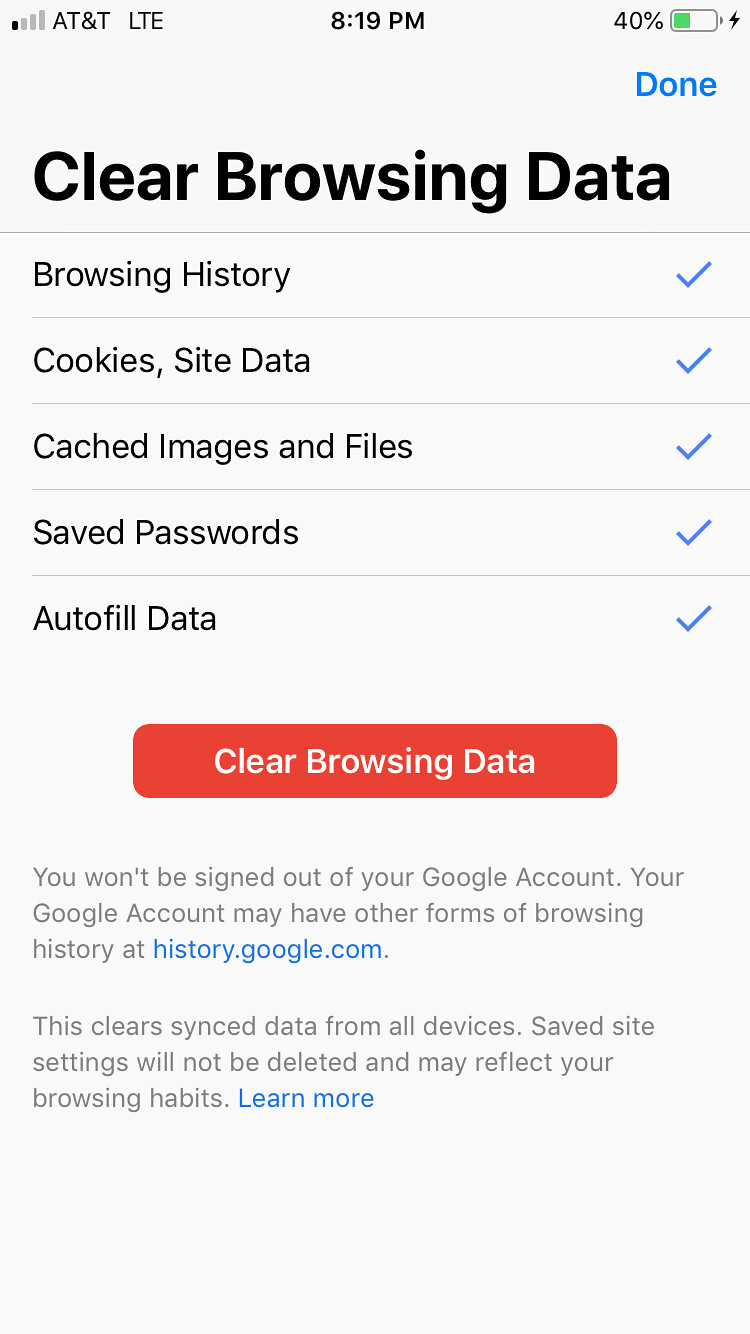The image depicts a screenshot of a Google Chrome browser on a cell phone, specifically showing the "Clear Browsing Data" screen. Prominently displayed at the top in black text is the title "Clear Browsing Data." Beneath this heading, a list of data types with corresponding blue checkmarks is highlighted, including "Browsing history," "Cookies and site data," "Cached images and files," "Saved passwords," and "Autofill data."

Centered below these options is a large red button with the text "CLEAR DATA" in white. Just underneath this button, a smaller gray text provides further explanation: "You won't be signed out of your Google account." It then explains that other forms of browsing history may exist on your Google account and directs users to "history.google.com" via a blue hyperlink. The text also states that "This clears sync data from all devices. Saved site settings will not be deleted and may reflect your browsing habits," followed by another blue hyperlink labeled "Learn more."

The overall background of this screen is gray. In the top left corner, signal bars and the service provider "AT&T LTE" are displayed. The time "8:19 p.m." is shown in the center of the top bar. To the top right, the battery status is indicated at 40%, represented by a partially filled green battery icon with a charging lightning bolt symbol. Directly below this battery icon, in blue text, the word "Done" is visible.